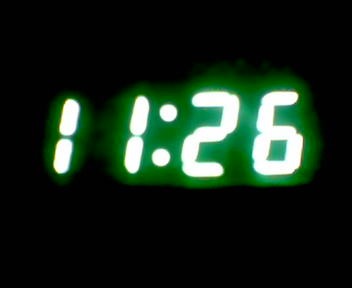The image depicts a glowing green digital clock displaying the time 11:26. The background is completely black, highlighting the bright LED digits. The numbers are constructed from individual segments: the ones are formed by two short segments stacked vertically, the two is made up of five segments, and the six uses six segments. The vivid green hue of the LEDs gives the numbers a distinct glowing effect, making them stand out starkly against the dark backdrop. The overall composition is minimalistic, focusing entirely on the luminescent green digits against the void of the black background.